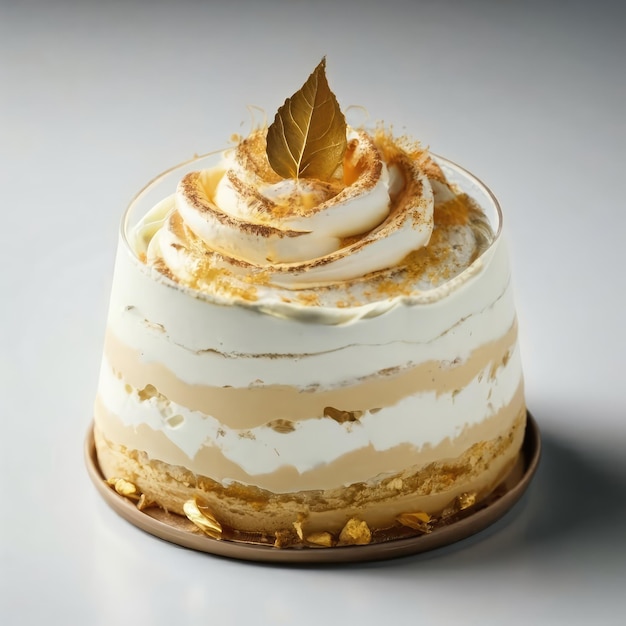In front of me is an elegant and refined dessert, presented in a clear cylindrical glass set atop a brownish golden saucer. The dessert features intricate swirled layers of creamy white whipped cream and beige pudding or caramel, resembling a trifle. The very top of the dessert showcases a delicate gold leaf garnishing the center of the swirls, with additional gold dust sprinkled over the cream. Small specks of gold leaf are also decoratively placed around the edge of the saucer. The entire setup is situated on a clear white surface, casting a subtle shadow beneath the glass. The sophisticated presentation and luxurious elements suggest this is an expensive dessert, suitable for festive occasions like fall or winter holidays. The background of the image is a smooth grayish white, enhancing the dessert's prominence.